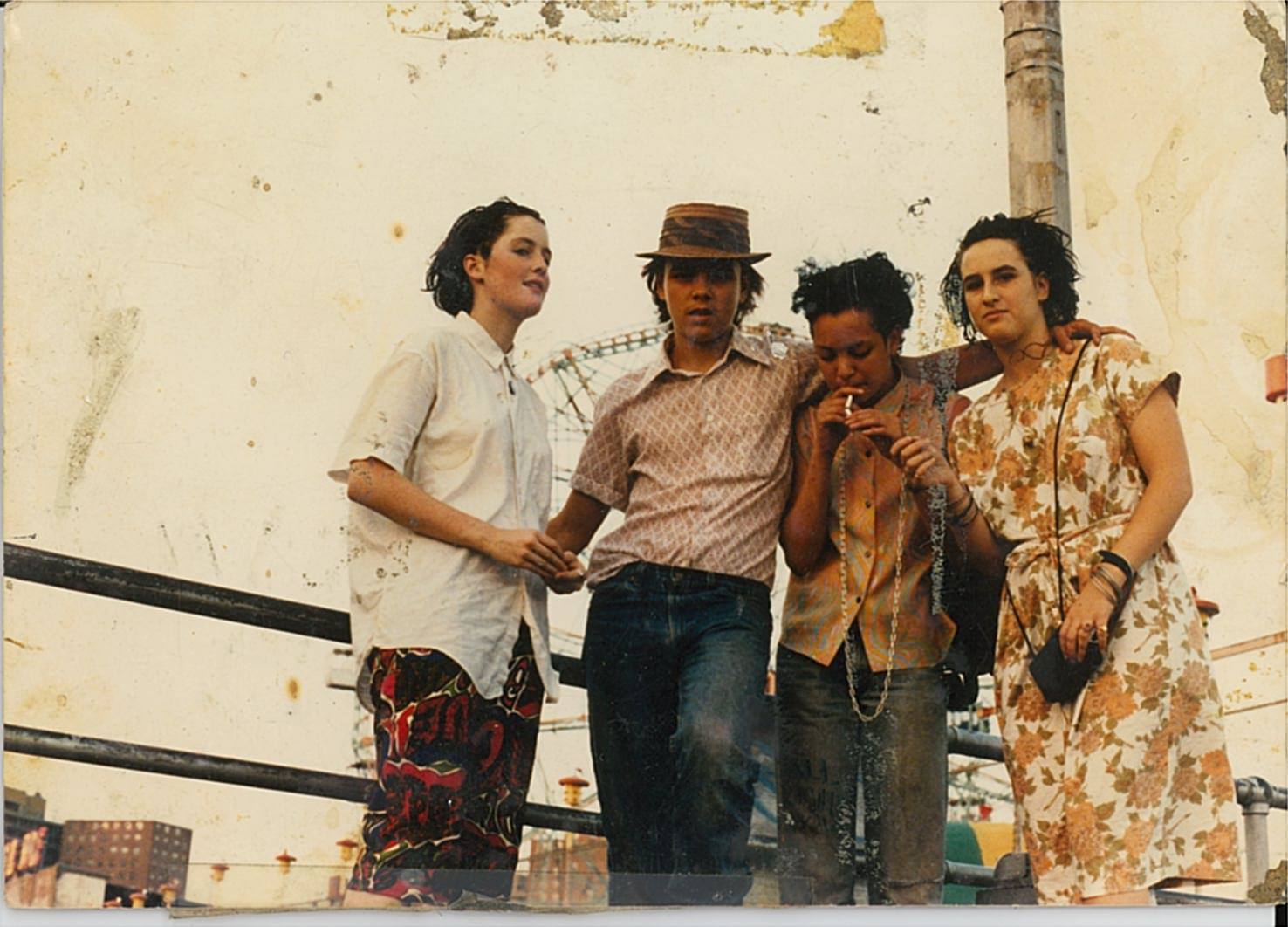This vintage photo captures a group of four young individuals standing atop a raised area, possibly a building, with a cityscape of apartment buildings in the backdrop. The image, weathered with visible cracks, breakage, and old adhesive markings, suggests it might have been taped somewhere once. The photo has faded over time, giving it a sepia or light yellow hue, adding to its nostalgic charm.

From left to right, the first individual is a Caucasian female with short black hair, dressed in a white short-sleeve top and black pants with red and white patterns. Next to her, an African-American male, sporting a brown fedora, wears a light brown and white cross-design button-up shirt and denim jeans. The third person appears to be an African-American woman lighting a cigarette; she is clad in a sleeveless, possibly orange-hued, button-up shirt paired with denim jeans and a long necklace. The final figure, whose gender is ambiguous, dons a large flower-patterned dress, jewelry, and has black hair.

In the background, two black metal horizontal bars suggest some form of railing, and a large Ferris wheel can also be discerned, hinting at a possible boardwalk or carnival setting. The overall appearance and ambient lighting suggest the photo was likely taken in the early evening.